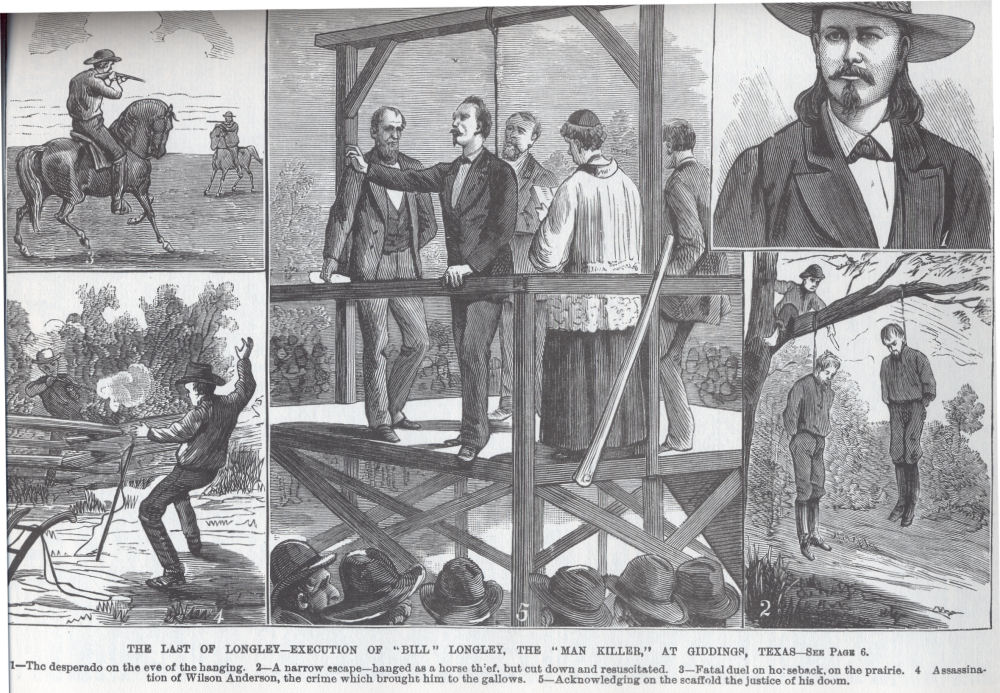The image is a detailed series of black-and-white pencil sketches depicting a dramatic Western scene, each section contributing to a somber narrative. In the top left sketch, two men on horseback aim rifles at each other, embodying the tense moments before a gunfight. Below, another drawing portrays a cowboy shooting at another across a fence, who is seen collapsing. In the center section, the focus shifts to a somber execution scene. Here, three men in suits and a clergyman stand by a man who appears to be uttering his last words on a platform with hanging ropes, surrounded by a crowd of onlookers, their hats and faces barely visible. To the side, a detailed portrait shows the same man in better times, dressed in a black jacket and hat. The final sections reveal a chilling conclusion: two men hanging from a tree with their hands tied and nooses around their necks, while another individual sits in the tree, appearing to adjust their positions.